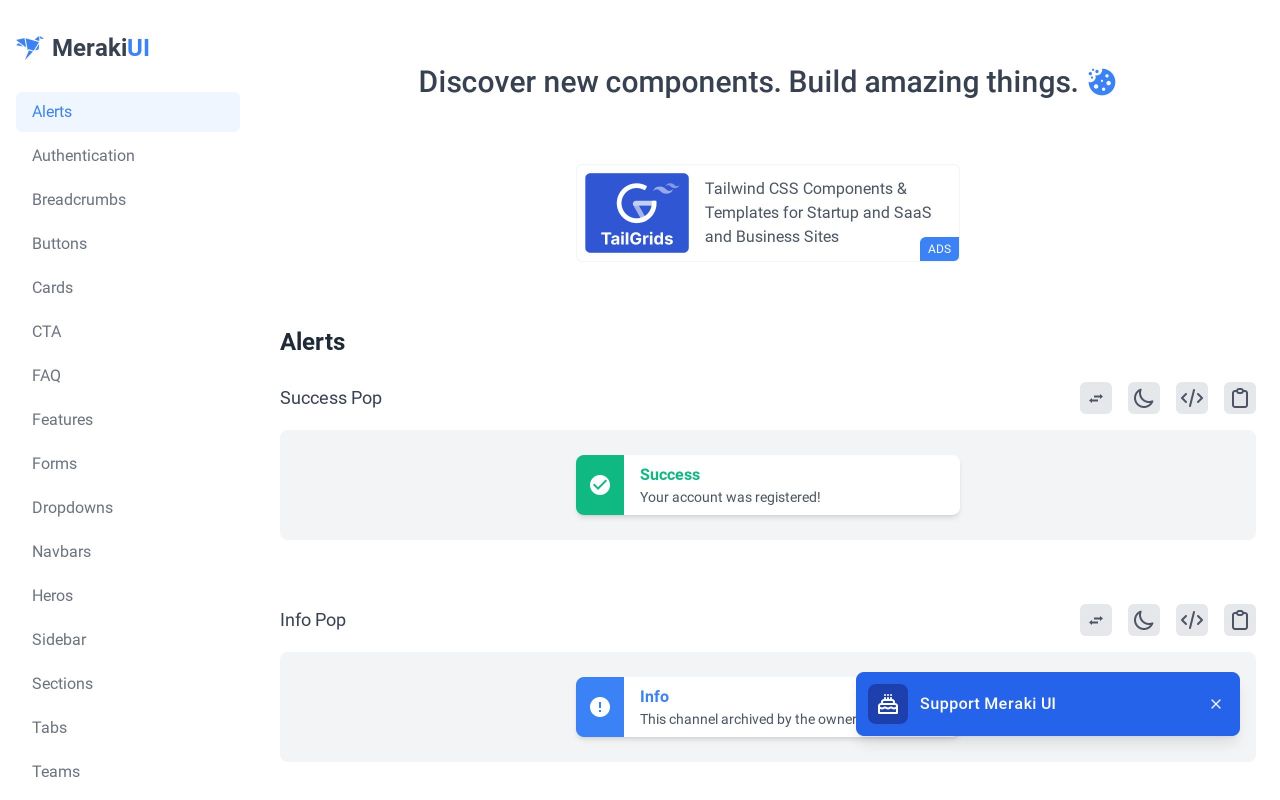This image from Merakai UI showcases a user-friendly interface designed to help you discover new components and build amazing projects. At the center of the image is the "Tail Grids" icon, prominently displayed in blue, accompanied by text explaining the available components and templates tailored for startups.

Beneath the central image, there are alert notifications that demonstrate the platform's messaging system. The first alert is a "Success Pop" message, featuring a long gray bar with a white interior that transitions into a green section with a check mark. This message reads: "Your account was registered." 

Below this, an "Info Pop" message is shown. It has a similar gray bar labeled "Info," which begins with the text "Support Merakai" followed by a truncated message ending with, "the channel activated by the..."

On the left side of the image, a sidebar lists various categories you can explore, including "Alerts," "Authorization," "Bread Buttons," "Cards," "CTA," "FAQs," "Features," "Forms," "Drop Downs," "Nav Bars," "Heroes," "Sidebar," "Sections," "Tabs," and "Teams," offering a comprehensive range of options for assistance and further functionality.